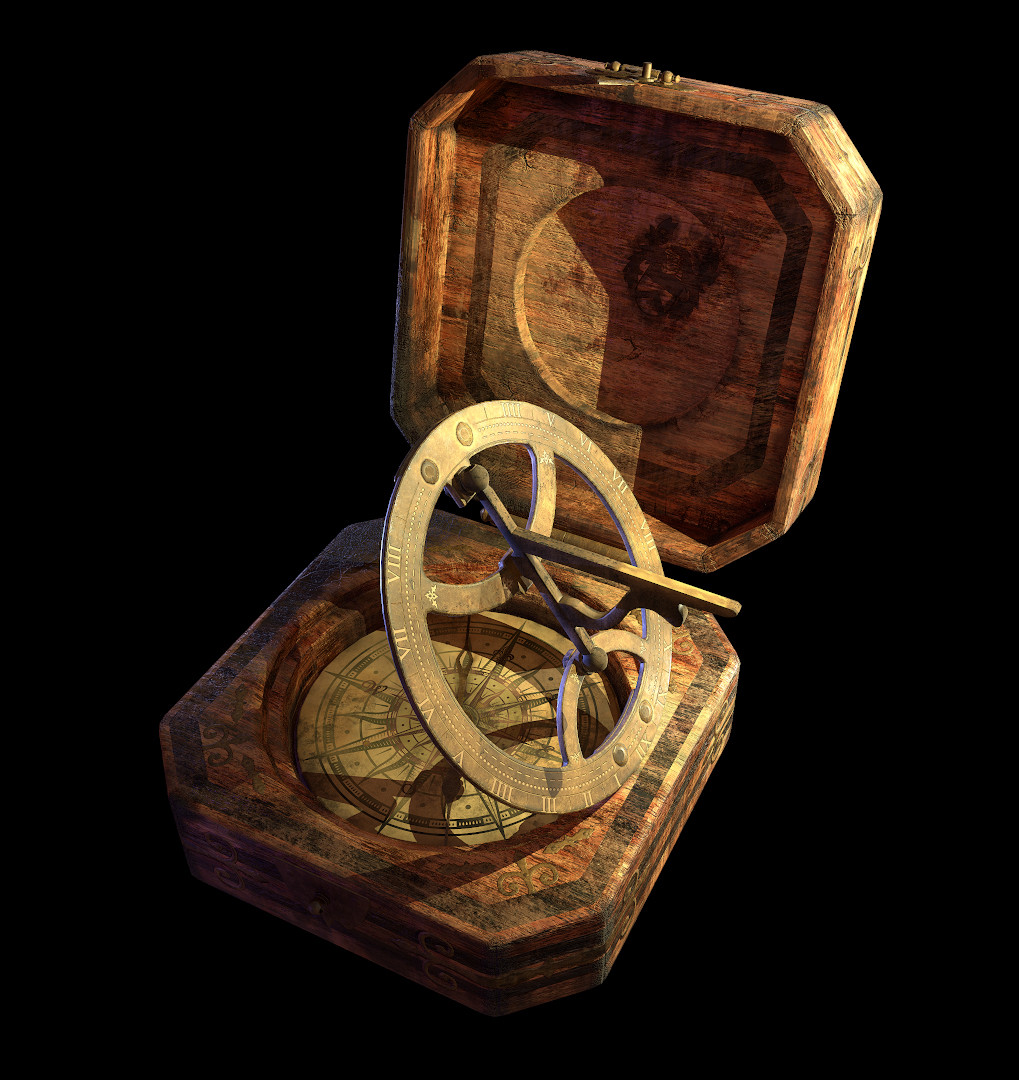The photograph, a vertically rectangular image with no border, depicts a meticulously staged scene using artificial lighting, albeit not very well-lit. Set against a deep black background, which gives the impression that the objects are floating, the focus is on an old, weathered wooden box with rounded edges and a gold latch. The box is distinctively open, revealing its contents. Inside, there is a hand-carved compass nested in the base of the box, showcasing intricate designs. Leaning against the compass and partially lifted out of the box is a brass sundial, identifiable by its Roman numerals and a protruding metal gnomon. The sundial, a glinting gold in color, casts a shadow to the left due to the light source coming from the right side of the frame. Both the compass and sundial exude a sense of antiquity, with the wood appearing faded and scratched, hinting at their long history.